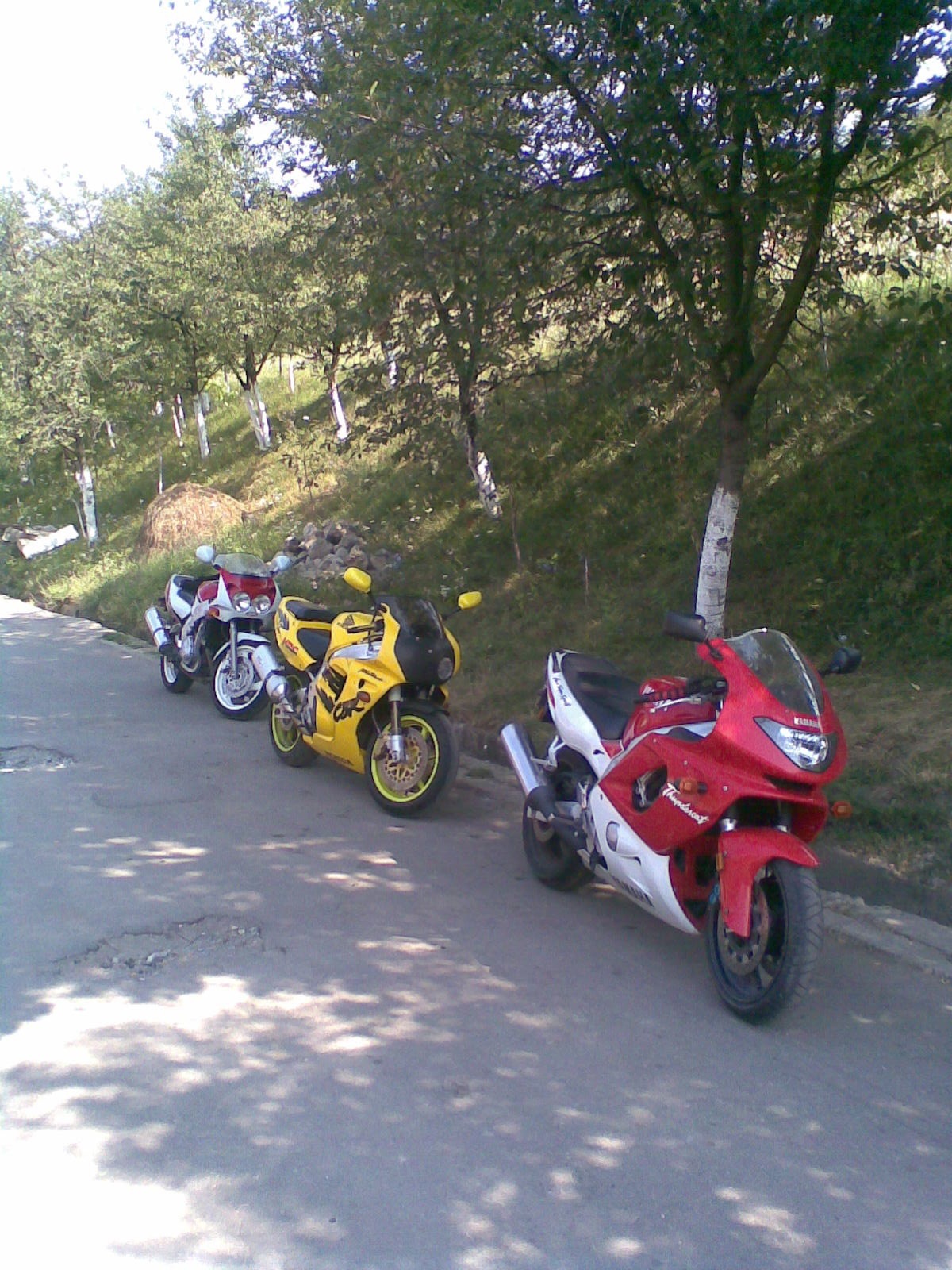This image features a light gray asphalt road peppered with potholes. To the right of the road, there is a steep, grass-covered hill dotted with numerous trees. Each tree has a white-painted base that transitions into its natural brown color partway up the trunk. Resting at the edge of the road are three Japanese-style motorcycles, all lined up and facing the same direction. The motorcycle closest to the foreground is red and white, the one in the middle is yellow and black, and the third motorcycle, like the first, is red and white. Further in the background, behind the motorcycles, there is a stack of hay, contributing to the rural scenery.